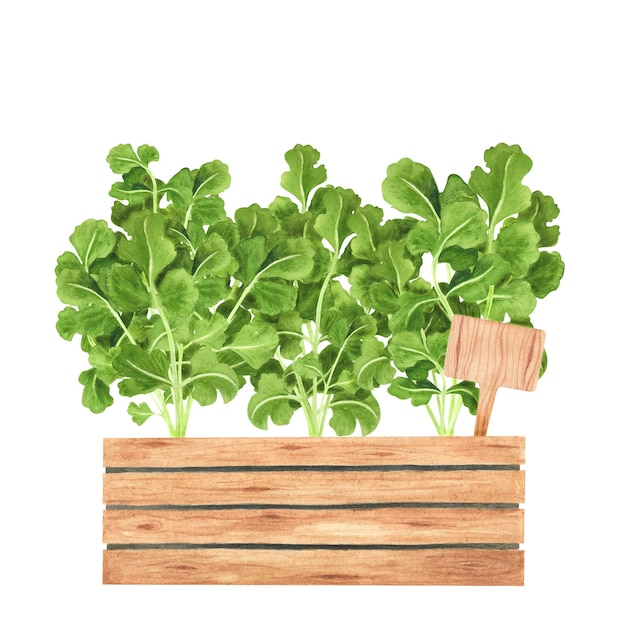The image depicts a flourishing sketch of a small herb garden cultivated in a wooden planter box. The box, natural in color and composed of four horizontal wooden slats, houses three clusters of identical green herbs. Each cluster is characterized by an abundance of lush, overlapping leaves with light pale green stems, giving the impression that the plants are still in their sprouting phase. There is a small wooden sign inserted in the right-hand side of the planter, intended for labeling the herbs, but it currently remains blank. The background of the image is white, drawing attention to the vibrant greenness of the herbs and the simplicity of the wooden planter.